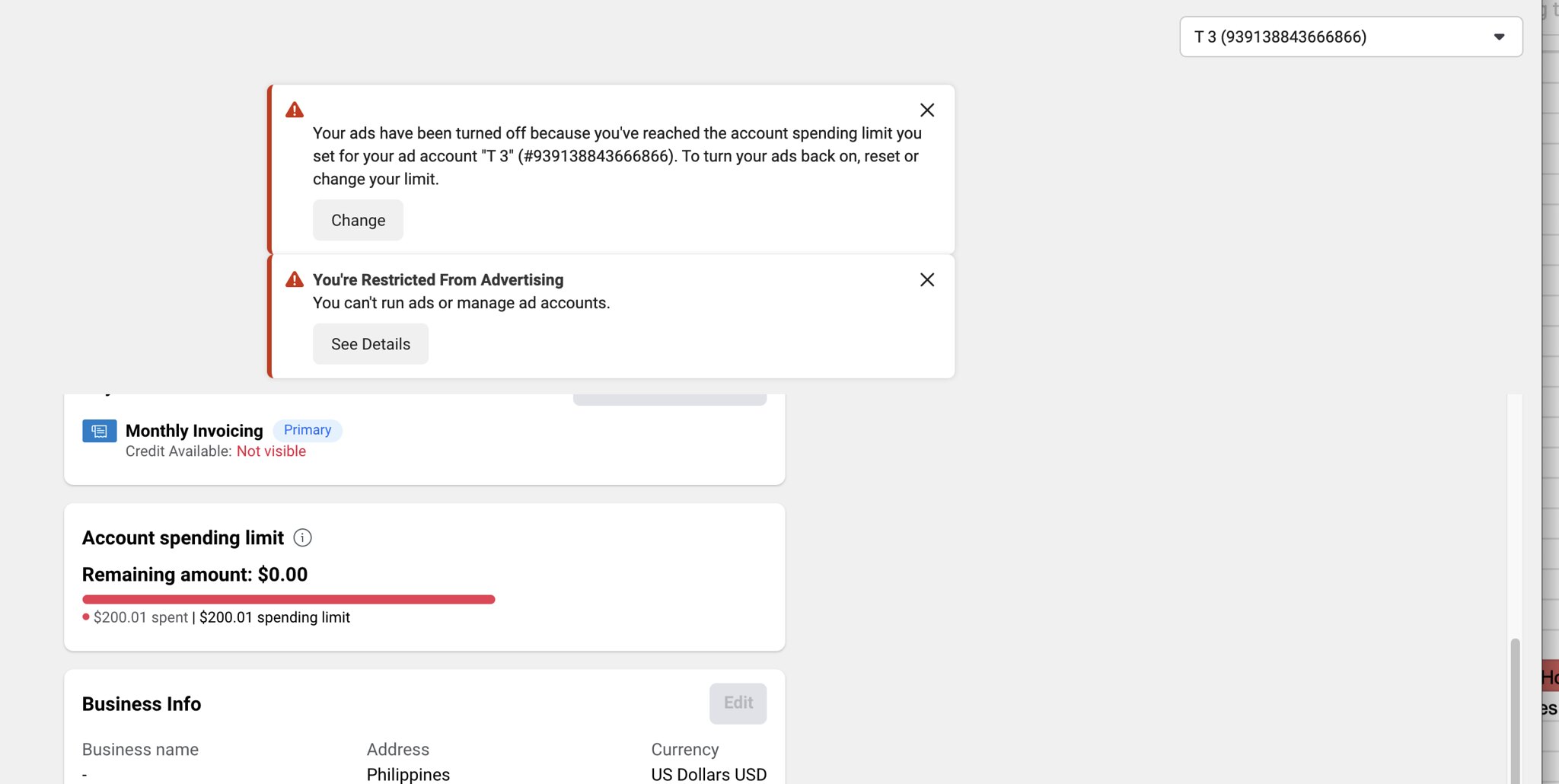This horizontal screenshot captures a section of an accounting or ad management software interface with a predominantly white background. In the upper right-hand corner, the screen displays "T3" followed by a long numerical sequence in parentheses and an inactive pull-down menu. 

At the upper center-left of the image, there’s a prominent rectangular alert box marked by red triangles featuring white exclamation points and 'X' icons for closing the window. The alert message reads:

"Your ads have been turned off because you've reached the account spending limit you set for your ad account T3, [followed by the same numerical sequence]. To turn your ads back on, reset or change your limit." Additionally, it states: "You're restricted from advertising. You can't run ads or manage ad accounts."

Below this alert box, to the bottom left of the image, there are three stacked rectangular sections with slight spacing between them. The top rectangle is a blue-colored box labeled "Monthly Invoicing Primary," with the phrase "Credit available not visible" in red. Below that, black text reads "Account Spending Limit," and it notes that the remaining amount is zero. A notable feature in this section is a horizontal red bar stretching from the left to just past the center, indicating "$201 spent, $201 spending limit."

The middle rectangle beneath this section is highlighted with bold black text saying "Business Info." It includes the details: "Business name, address, and currency," indicating that the business name is not displayed, the address is listed as the Philippines, and the currency used is U.S. dollars.